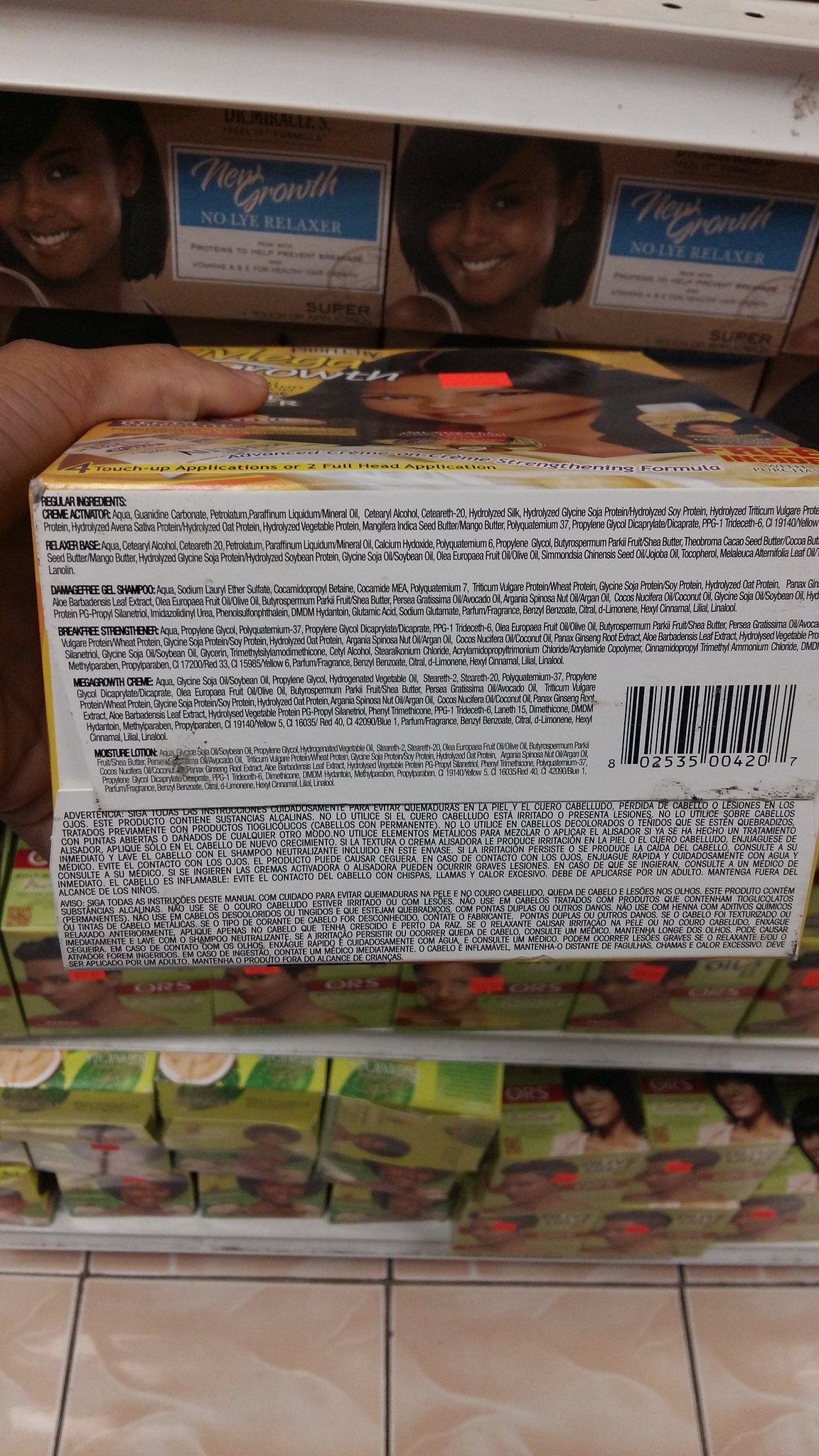This image captures an aisle in a beauty supply or health and beauty store, showcasing a vibrant display of women's hair care products. Prominently, we see a yellow box of "New Growth No Lie Relaxer" featuring an African-American woman with black hair on the front. A person is holding this box, revealing the UPC code, usage instructions, and ingredients. The box also has a red sticker, indicating it might be marked down. Below, two more shelves are filled with additional hair care products, many of which also bear red sale stickers, suggesting a broader markdown event. The bottom shelf contains green packages, each featuring an African-American woman on the cover. The entire scene is set against a backdrop of beige, grocery store-style tile flooring.